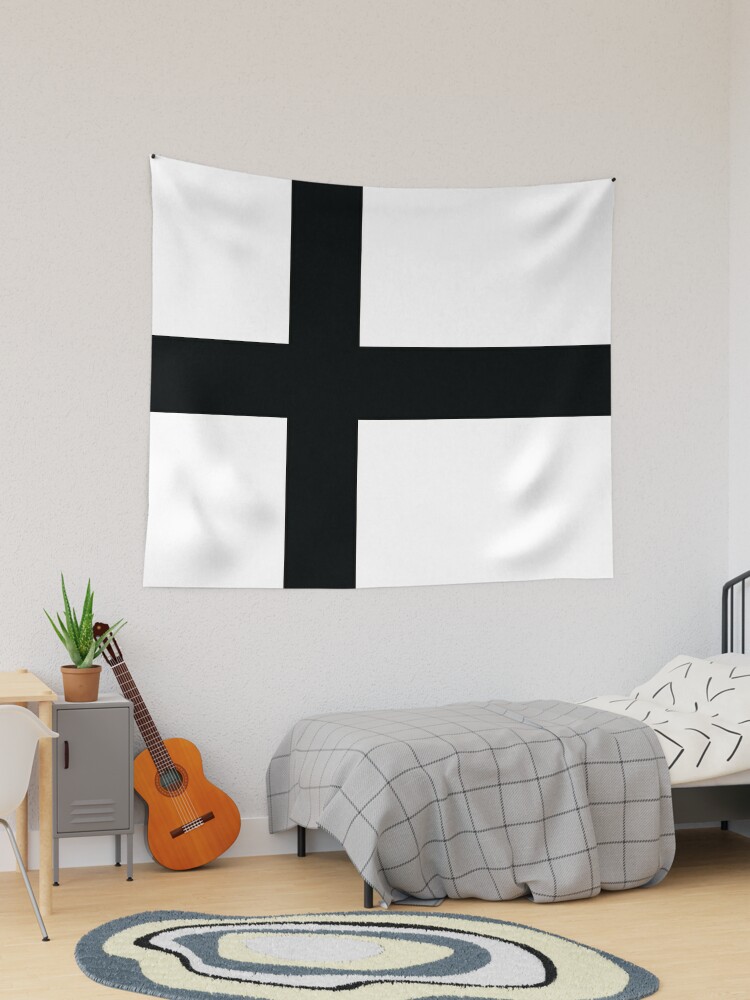This color photograph depicts a meticulously arranged kid's bedroom with light oak or pine wood flooring. The room features a striking decor element: a large white flag tacked to the wall, adorned with a black cross. The bed below, with its iron frame and gray comforter, is complemented by a white and black checkered sheet set. A modern Scandinavian-style area rug lies in front of the bed, showcasing amoeba-like, wavy concentric circles in shades of gray, yellow, blue, black, and white. To the side, a compact, gray locker serves as a nightstand, topped with a potted aloe vera plant. A brown acoustic guitar leans diagonally against the locker. The partially visible pine-colored desk suggests a neat yet creative space for a child.